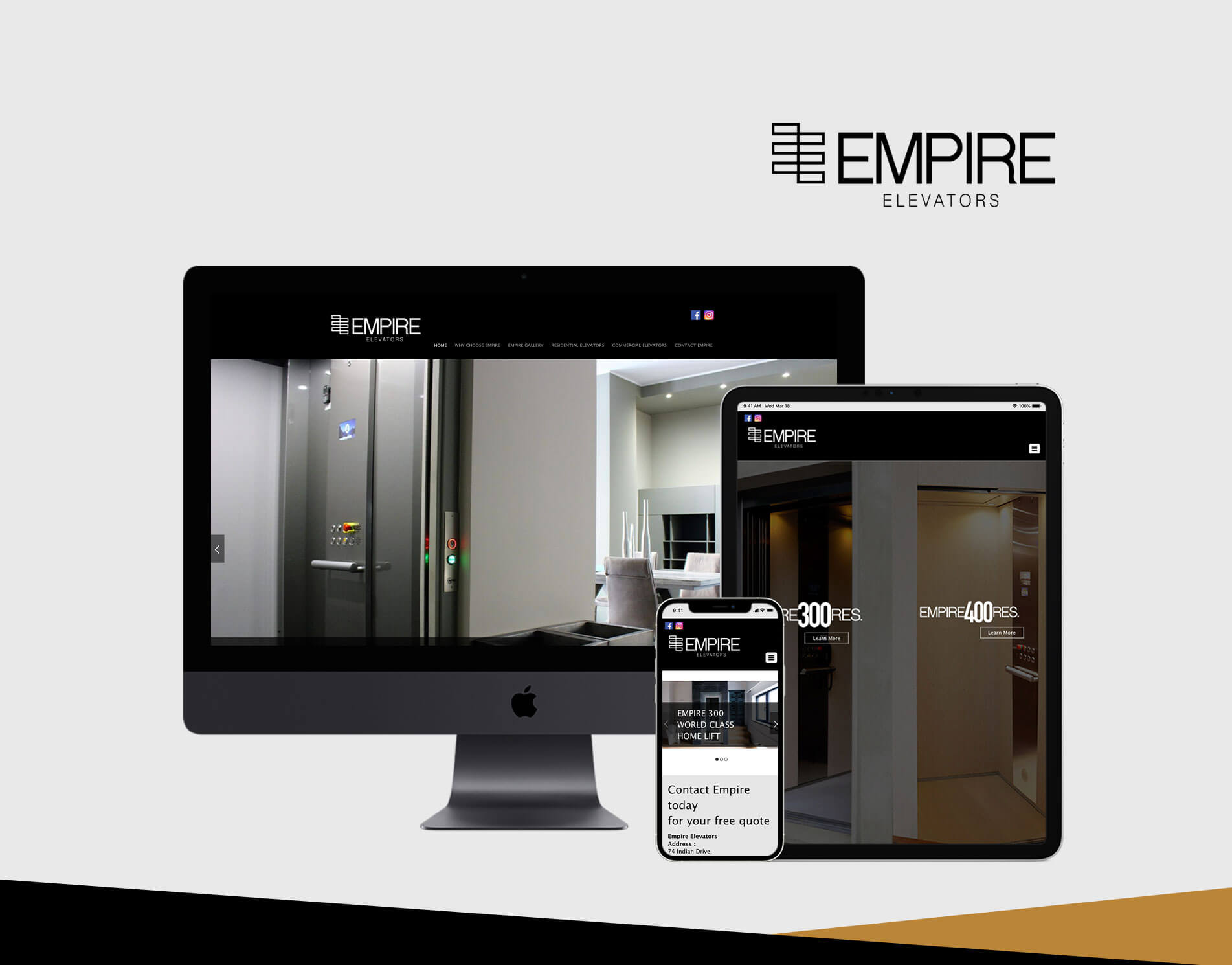This advertisement for Empire Elevators features a sleek, technology-themed layout set against a predominantly white, light gray background, accented by a thin black and gold border at the very bottom. Dominating the center of the image is an Apple computer monitor displaying a high-resolution image of the inside of a silver elevator, complete with visible buttons and a handle. To the left of the monitor, a silver elevator door enhances the modern aesthetic. 

In front of the monitor, an Apple iPad and an Apple iPhone are arranged with precision. The iPad, positioned slightly forward, mirrors the elevator image shown on the monitor, encapsulating the detailed view of the elevator door and controls. The iPhone, placed at the front, prominently showcases the Empire logo at the top, with the message "Empire 300 World Class Home Lift" in the center, and "Contact Empire today for your free quote" at the bottom, reinforcing the call to action. 

The upper right corner of the image features the bold black text "Empire Elevators," accompanied by the company's logo, anchoring the ad with a professional touch. Subtle hints of a home setting, perhaps a dining room table or window, provide an inviting atmosphere that highlights the elevator's integration into everyday life. The cohesive color scheme of black, white, tan, and silver exudes elegance and reliability, making this ad a compelling invitation to modernize one's living space with Empire Elevators.